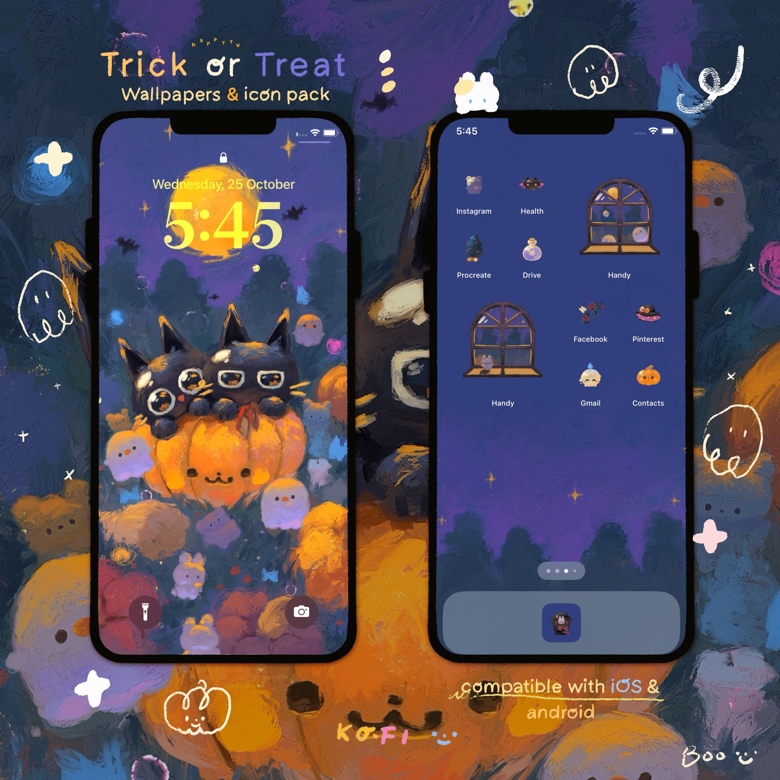In this detailed image, two main sections draw immediate attention: the left and the right, each displaying a phone screen against a vibrant, well-crafted painting as the backdrop. At the bottom of the composition, a whimsical, Halloween-themed illustration features a cat perched atop a carved pumpkin, enhancing the seasonal atmosphere.

The top left corner of the image prominently displays the words "Trick or Treat, Wallpapers and Icon Pack." Below this header, the phone screen on the left showcases a status bar at the top middle indicating "Wednesday, 25 October, 5:45." The battery icon on the top right corner of the phone is fully charged, and the WiFi signal strength is maxed out, ensuring connectivity. The bottom corners of this phone screen include a flashlight icon on the left and a camera icon on the right, hinting at quick access functionalities. 

On the right-side phone screen, a grid of various app icons is visible. "Instagram" occupies the top left, with "Health" immediately to the right. Below "Health," the "Drive" app is displayed, and to its left, the "Procreate" app. At the top right is the "Handy" app, followed by "Facebook," "Pinterest," "Gmail," and "Context" below it. The "Context" app is visually represented by a pumpkin icon, while the "Gmail" app icon is styled to resemble a knight.

In the lower right corner of the full image, the words "Boo" with a smiley face add a playful touch. To the left of this, text confirms compatibility with both iOS and Android platforms. This descriptive scene combines elements of functionality with a festive Halloween spirit.